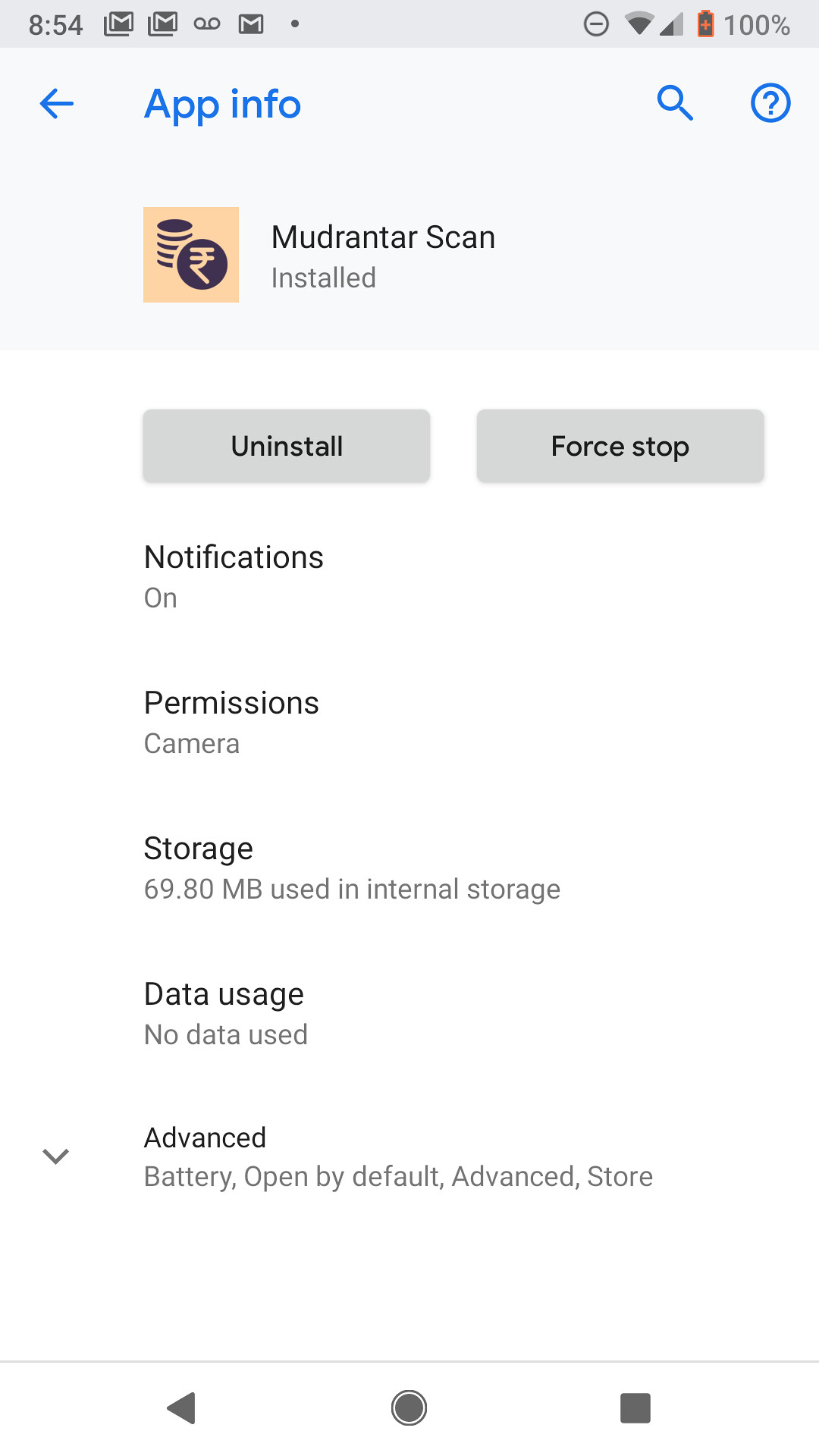This image is a screenshot of the "Mudrantar Scan" mobile application displayed in vertical portrait mode on a smartphone. The screen, titled "App Info" in blue text with a left-pointing arrow beside it for navigation, provides detailed information about the app. A peach-colored square icon featuring a stack of round black coins and a vertically positioned black coin with a foreign symbol (possibly Chinese or Japanese) is positioned to the left of the app's title. 

On the upper right corner, there are two icons: a magnifying glass representing search functionality and a question mark for help or additional information. Below the app's name, two gray buttons labeled "Uninstall" and "Force Stop" allow the user to manage the app.

The detailed information section lists:
- Notifications: On
- Permissions: Camera, Storage 
- Storage: 69.80 MB used in internal storage
- Data Usage: No data used
- Advanced sections for Battery and Opening by Default

At the bottom of the screen, the photograph also captures part of the device’s recording interface, which includes a left-facing triangle for play, a round button for starting and stopping recording, and a square button for stopping.

The background of the screen is predominantly white, with a light gray banner at the top where the app’s name and navigation elements are located.